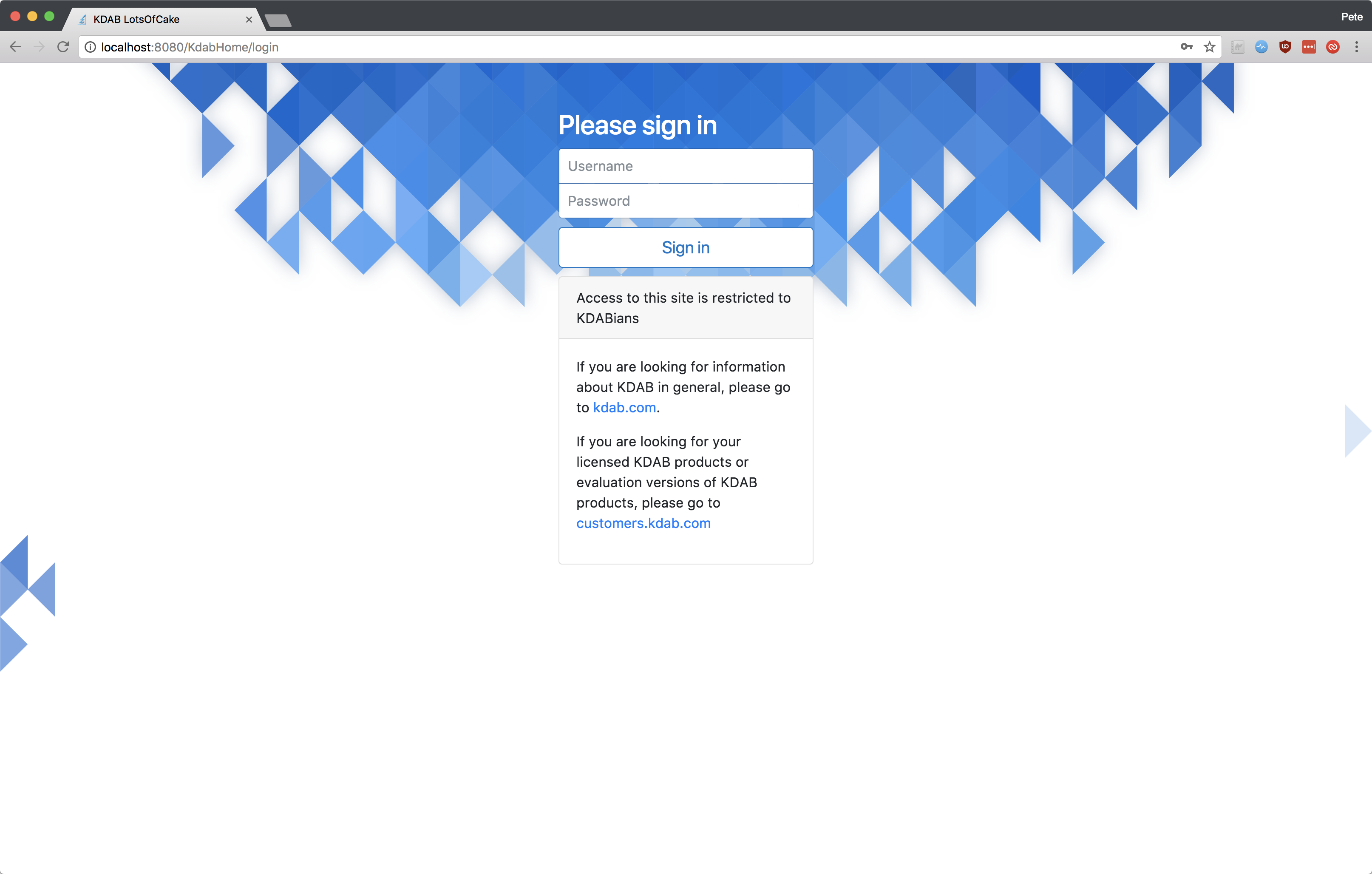**Descriptive Caption:**

The image displays a web browser tab with the title "KDAB - Lots of Cake," showing the URL "http://localhost:8080/KDAB/home/login". The webpage features a quilt-like background with interlocking blue diamond shapes forming a V-pattern that descends from the top edges to the center of the page. At the center of this V is the text "Please Sign In" in white font against the blue backdrop.

Below this text, there are two data fields labeled "Username" and "Password," both outlined in white. A matching white button with the text "Sign In" in blue is positioned directly beneath the fields. Additional informational text indicates that access to the site is restricted to "KDABIANS," and provides instructions for those seeking general information or product licenses to visit "KDAB.com" or "customers.kdab.com" respectively.

The overall color scheme of the webpage includes blue, white, gray, black, with accents of red, yellow, green, and orange. In the browser interface, there is a black bar behind the open tabs, adding to the visual structure on the right side of the screen.